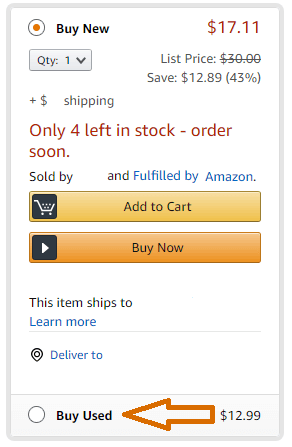The image depicts a zoomed-in view of a product purchasing page on the Amazon app or website, specifically showing detailed information about buying the product new or used. The product has a new purchase price of $17.11, which is down from a list price of $30—a 43% discount, saving the buyer $12.89. Currently, only four units are left in stock, indicated by a prompt urging to "order soon." This product is sold and fulfilled by Amazon.

The page features two prominent action buttons: a dark yellow "Add to Cart" button with a cart symbol and an orange "Buy Now" button with a play symbol. Below these buttons, there is information saying "This item ships to [destination]," with a clickable "learn more" link in blue font. Additionally, there is a "Deliver to" link in blue font, also clickable.

Lastly, the section for buying the product used is highlighted with an orange arrow pointing to the word "used," indicating it is available for $12.99.